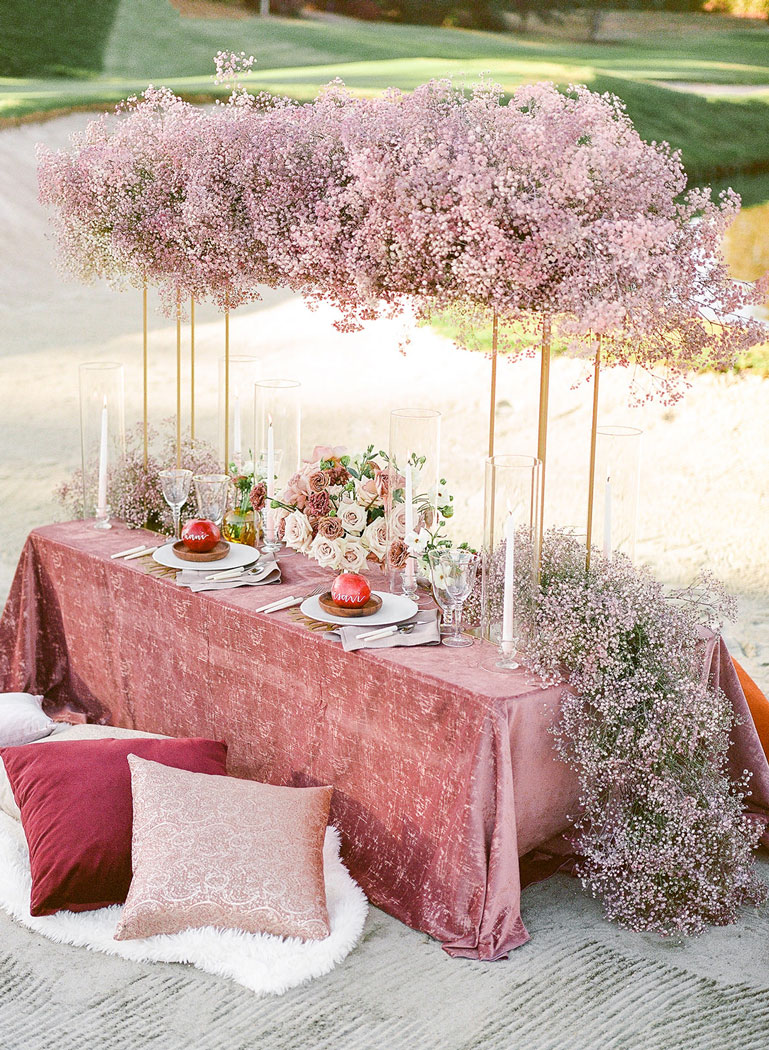Set in the middle of a sandy field or a sand trap on a golf course, this photograph captures an elegantly arranged dining table, perfect for a romantic occasion. The long, square table is draped in an ornate mauve pink velvet tablecloth that flows all the way down to touch the sand. In front of the table lies a luxurious white fur rug adorned with pillows in hues of red, yellow, and burgundy.

The table is meticulously set for two, featuring white plates paired with smaller gold ones, each cradling a pomegranate. White-handled cutlery and mauve pink napkins accompany each setting, while crystal water and wine goblets stand next to the plates. Multiple candles in crystal jars add a warm glow to the arrangement, enhancing the romantic ambiance.

The centerpiece of the table is a stunning bouquet of roses in shades of pale pink, deep mauve, and red, complemented by delicately dyed pink and mauve baby's breath. This floral theme extends upwards into a canopy-like structure formed by a trellis adorned with the same soft, tiny pink flowers, creating an enchanting overhead display. The scene is set against the contrasting backdrop of the lush green golf course, making it a picturesque and dreamy dining setup.